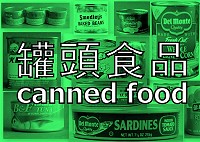Caption: 
This green-tinted collage features an array of 11 different types of canned foods meticulously arranged across the image. The centerpiece contains white text with black outlines, displaying Chinese writing. In the upper right corner, a Del Monte can is prominently showcased. The bottom section includes a can of sardines, standing out amidst the other canned items. On the upper left, three distinct cans can be observed, contributing to the diverse assortment. The green filter casts a uniform hue over the entire image, creating a cohesive and visually appealing presentation of the various canned goods.